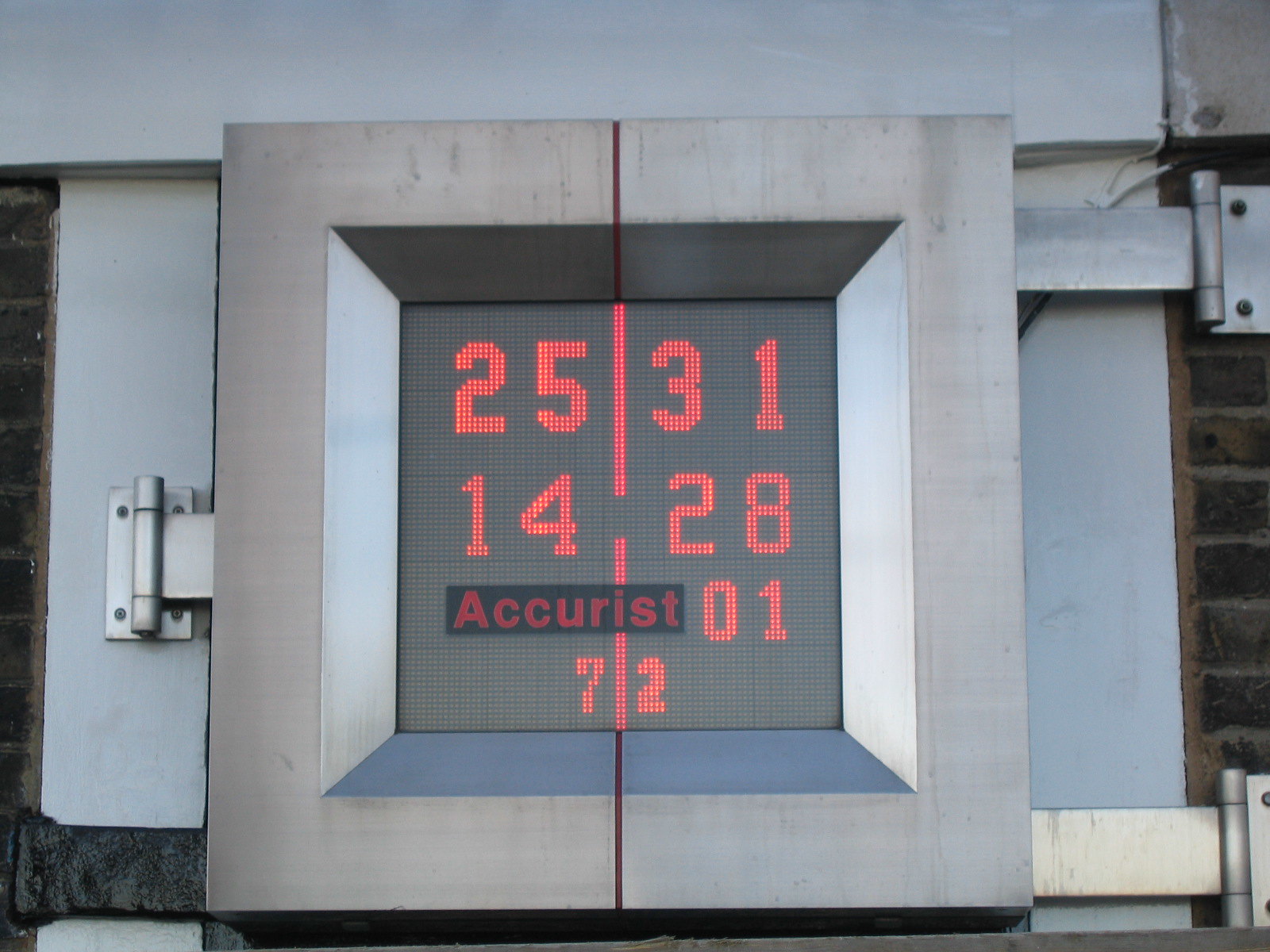A digital device, resembling a small safe, is mounted on a black brick wall. The device is secured to the wall with three silver brackets—two on the right side and one on the left. The body of the device is silver and square-shaped, with a black background that highlights its digital display. The red digital numbers read: 25, 31, 14, 28, 01, and 72. Cutting through the middle of the display is a horizontal red line. Below the numbers, a black rectangular panel features the word "Accurist" in red letters. Additionally, a wire emerges from the right corner of the square device, adding to its industrial look.